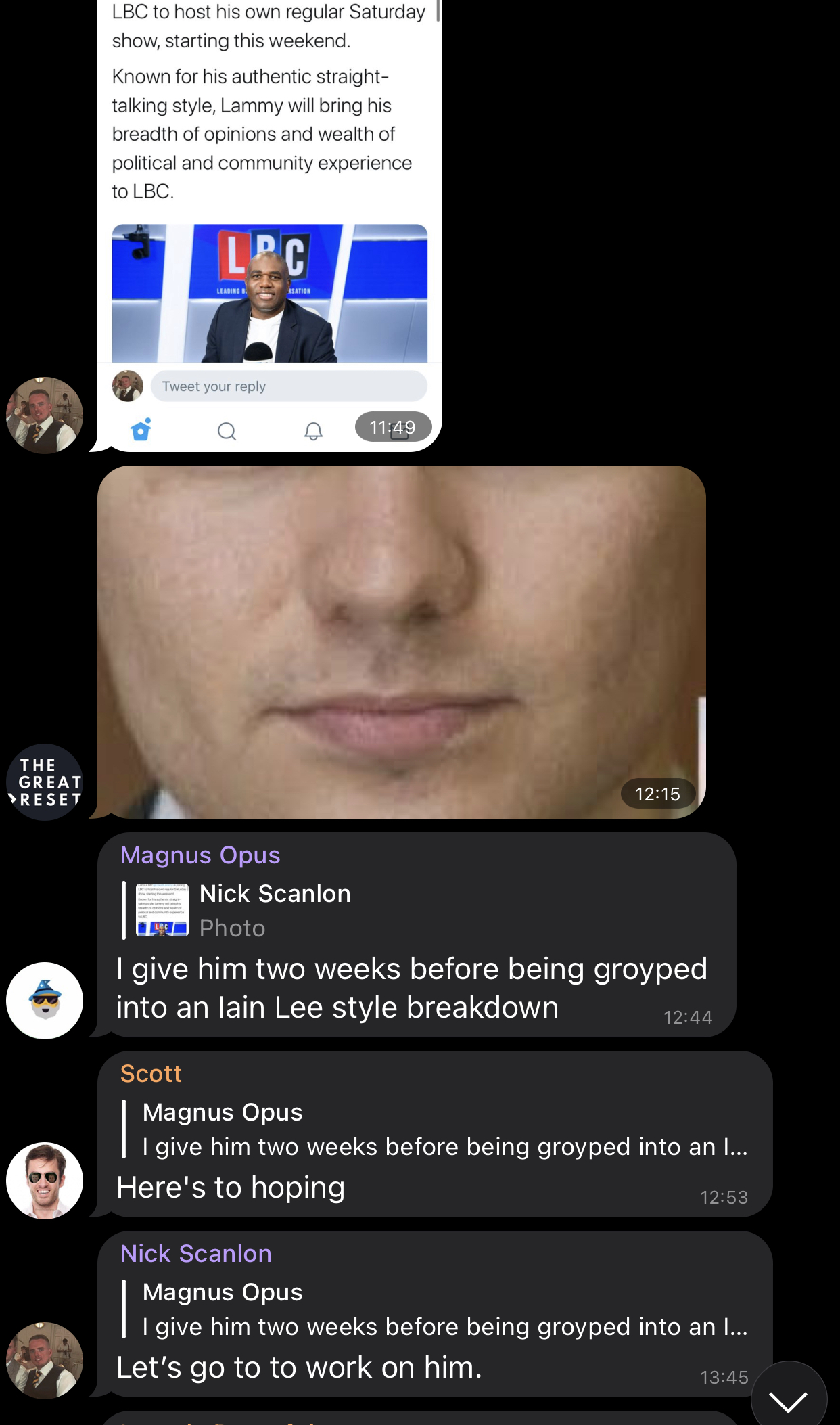This image is a screenshot taken from someone's cell phone, displaying a chat from an application. At the top of the screen, a speech bubble appears next to a user's profile picture, announcing, "LBC to host his own regular Saturday show starting this weekend. Known for his authentic, straight-talking style, Lammy will bring his breadth of opinions and wealth of political and community experience to LBC." The top right corner shows the time, 11:49.

As the conversation continues, the bottom of the image captures only the nose and mouth of another user. Below that, a message reads: "The Great Reset." User Magnus Opus comments, "I give him two weeks before being groyped into a Lane Lee-style breakdown." Scott responds with, "Here’s to hoping," followed by Nick Scallion's comment, "Let's go to work on him."

The entire background is black, with the chat conversation predominantly occurring on the left side of the screen, though it disperses to the right as more users reply to Magnus Opus. Other users' profile pictures and messages are visible, contributing to the ongoing discussion.